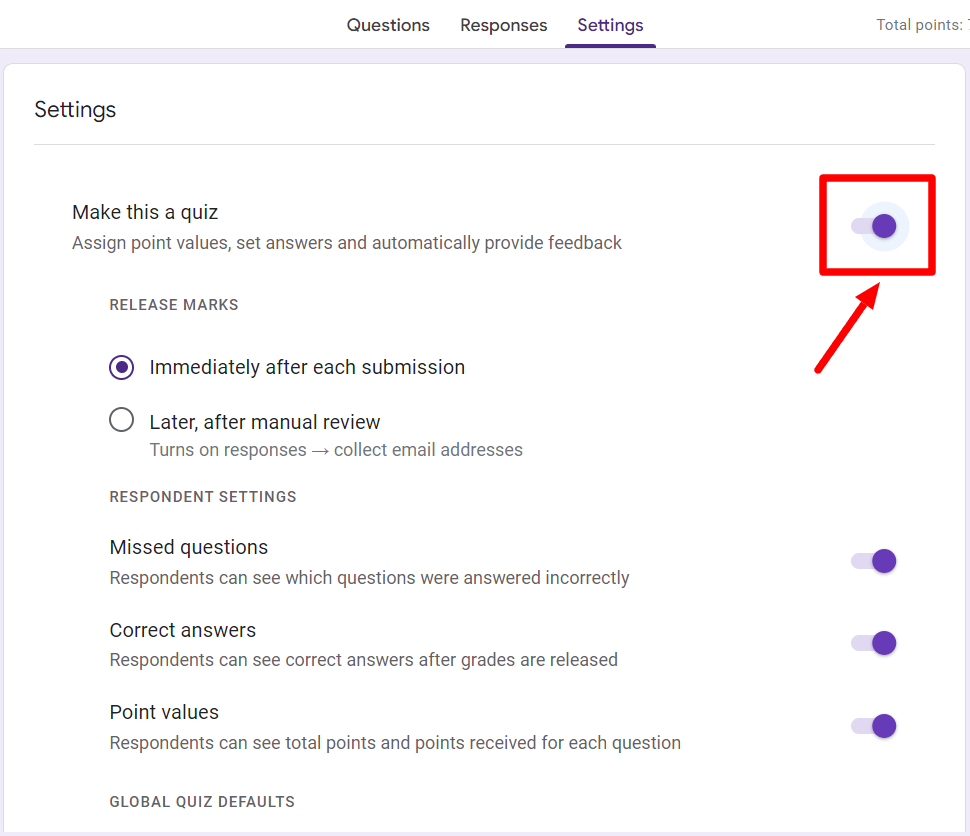This image captures a detailed view of the "Settings" tab of a computer screen, specifically within a quiz application. At the top of the screen, the tabs "Questions," "Responses," and "Settings" are visible, with "Settings" highlighted and underlined to indicate the active tab. On the right side, there is a label "Total points" displayed without any corresponding values.

The "Settings" tab presents several options for configuring the quiz:

1. **Make this a quiz:** This feature is highlighted with a large red box and an arrow pointing to it, indicating that it is currently enabled. It allows for the assignment of point values, setting of correct answers, and the provision of automatic feedback.

2. **Release marks:** This dropdown menu offers two options for releasing quiz results. The currently selected option is "Immediately after each submission." The alternative choice, "Later, after manual review," is not selected.

3. **Collect email addresses:** This option is switched on, as indicated by the active toggle switch.

4. **Respondent settings:** All features under this section are enabled, marked by dark purple toggles to the right-hand side:
   - **Missed questions:** Respondents can see which questions were answered incorrectly.
   - **Correct answers:** Respondents can see correct answers after grades are released.
   - **Point values:** Respondents can see total points and the points received for each question.

At the bottom of the visible section, the text "Global quiz defaults" is noted, but the page cuts off before providing further information.